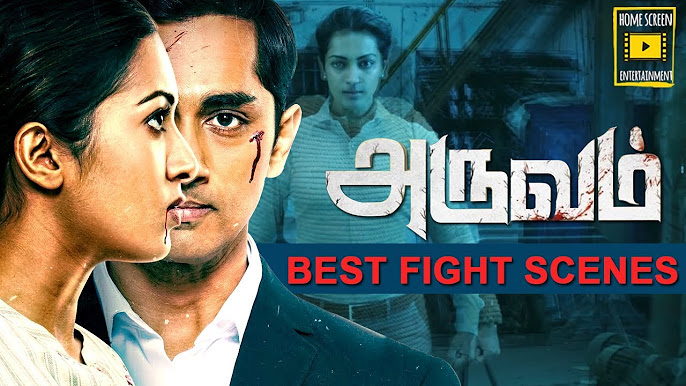The image appears to be a promotional cover for a TV show or movie, featuring a dramatic and intense scene with a blue-tinted background. On the left-hand side, we see the side profile of a Southeast Asian woman, possibly Indian, wearing a white shirt, with blood trickling from the right side of her mouth. Behind her is an Indian man, seen from the shoulders up, wearing a white collared shirt under a black blazer. He has visible cuts with blood on his cheek and forehead. 

In the background, the same woman is depicted from the front, her hands clenched into fists, suggesting she is ready to fight. She looks determined and battered, hinting at a physical struggle. This background image is tinted blue and looks like it could be a scene from a movie.

At the top right corner, there is a yellow-bordered logo with white text that reads "Home Screen Entertainment," and features a yellow play button icon. Below this, centered in the image, white text with blood splatters—written in a foreign language, potentially Hindi—precedes bold red capital letters that state "Best Fight Scenes." The overall aesthetic of the image suggests it is an advertisement for action-packed content focused on intense fight sequences.